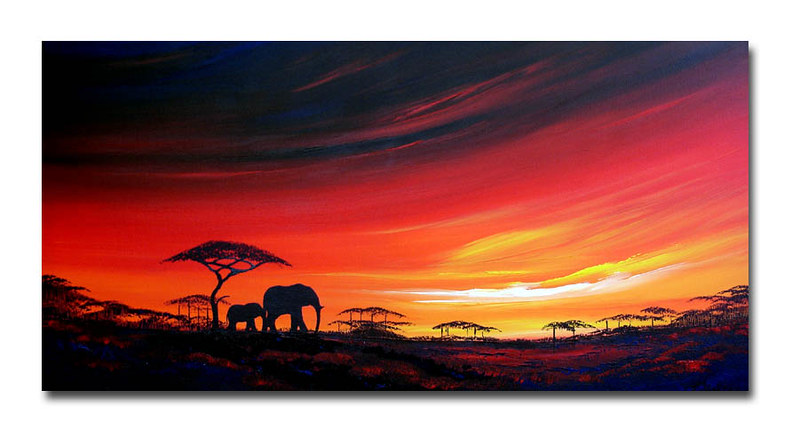This is a horizontally aligned rectangular oil painting without a border. At the top-left corner, the sky starts as a dark black that transitions into various shades of blue, mingling with pink towards the right, creating a dawn or dusk effect. The middle section features striking stripes of red and pink, shifting to vibrant bands of yellow and orange lower down, indicative of a vivid sunrise or sunset. A prominent, bright white strip in the lower right suggests the hidden sun illuminating the sky behind it. 

The bottom 20% of the painting depicts a dark, almost silhouetted landscape, likely representing a Sub-Saharan African scene. Scattered trees punctuate the land; these trees have slim trunks with broad, umbrella-like tops. On the lower left, the silhouettes of two elephants—a larger one followed by a smaller one, both facing left to right—stand between the trees. These animal shapes are simply rendered in black, highlighting their presence against the colorful sky.